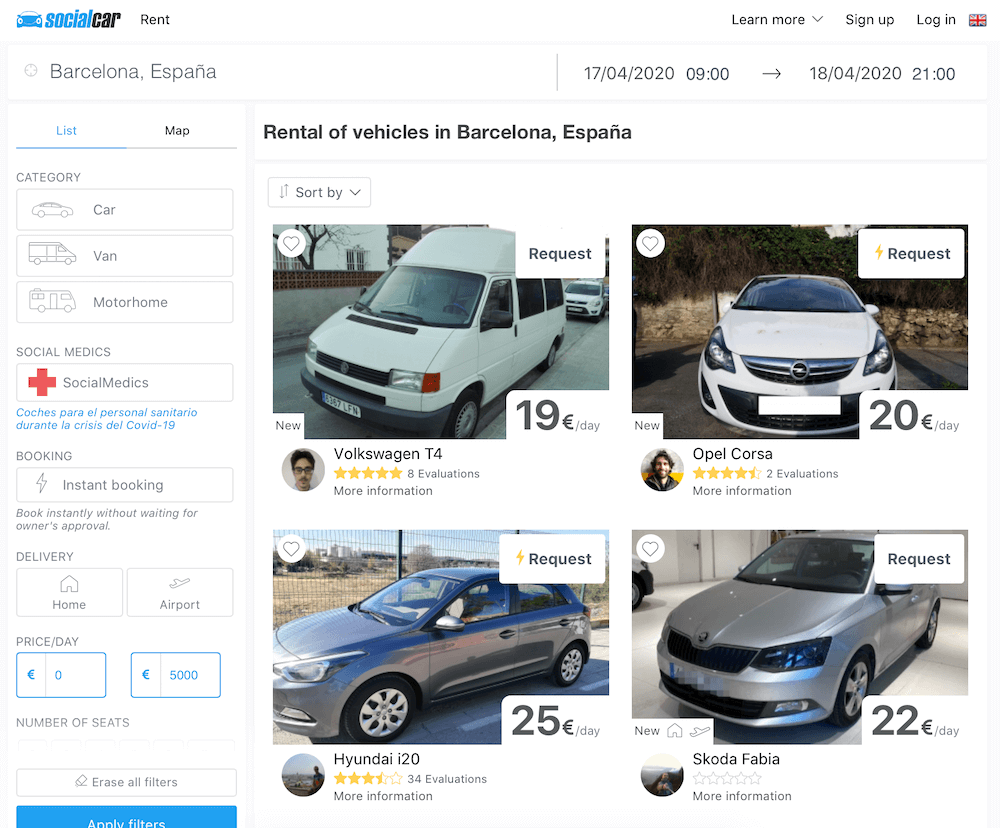**Detailed Caption of a Motor Vehicle Rental Web Page:**

This image captures a screenshot of a motor vehicle rental web page. The background is predominantly white, offering a clean and user-friendly appearance. At the very top of the page, the company’s branding is presented with a blue accent. The logo features a digitally illustrated front view of a sports car, primarily in blue. The company name is displayed with "Social" in blue and "Car" in bold black, followed by a space and the word "Rent."

Below the logo, there is a search box accompanied by an icon of a magnifying glass. The search input field is pre-filled with "Barcelona, Espana," indicating Barcelona, Spain. To the right of this search box, there are date and time selectors for the rental period. The first set shows "17th April 2020, 9:00" and an arrow pointing to the right indicating the end date, which is "18th April 2020, 21:00."

To the left of the search box, there are two clickable options: "List," which is highlighted in blue, and "Map." Below this toolbar, a category selection box is displayed with icons and options for different types of vehicles, including a car, van, and motorhome, each depicted by a side view illustration.

Further down, there is a section titled "Social Medics" featuring a red cross symbol, indicating a likely reference to the medical community. Accompanying this are Spanish text details below it. The next segment includes a "Booking" option with an instant booking feature highlighted by a lightning bolt icon. The description specifies "Book Instantly, Waiting for Owner's Approval." This section uses a lighter gray color with a thinner font for a more subdued appearance.

Underneath the booking section, there are icons for "Delivery" options with illustrations of a house and an airplane, indicating home and airport delivery options respectively. Following this is the "Price and Day" section showcasing two blue boxes displaying rates in a foreign currency, suggested to be liras or another non-dollar currency.

Centrally located on the page, in a dark bold font, the heading "Rental of Vehicles in Barcelona" captures the user’s attention. Below this heading, there are four images arranged in a two-by-two grid, showing front and side views of four different cars: a Volkswagen, a Corsa, a Hyundai i20, and a Skoda Fabia. Each car listing includes the name of the person offering the vehicle, a five out of five stars rating system, and the daily rental price.